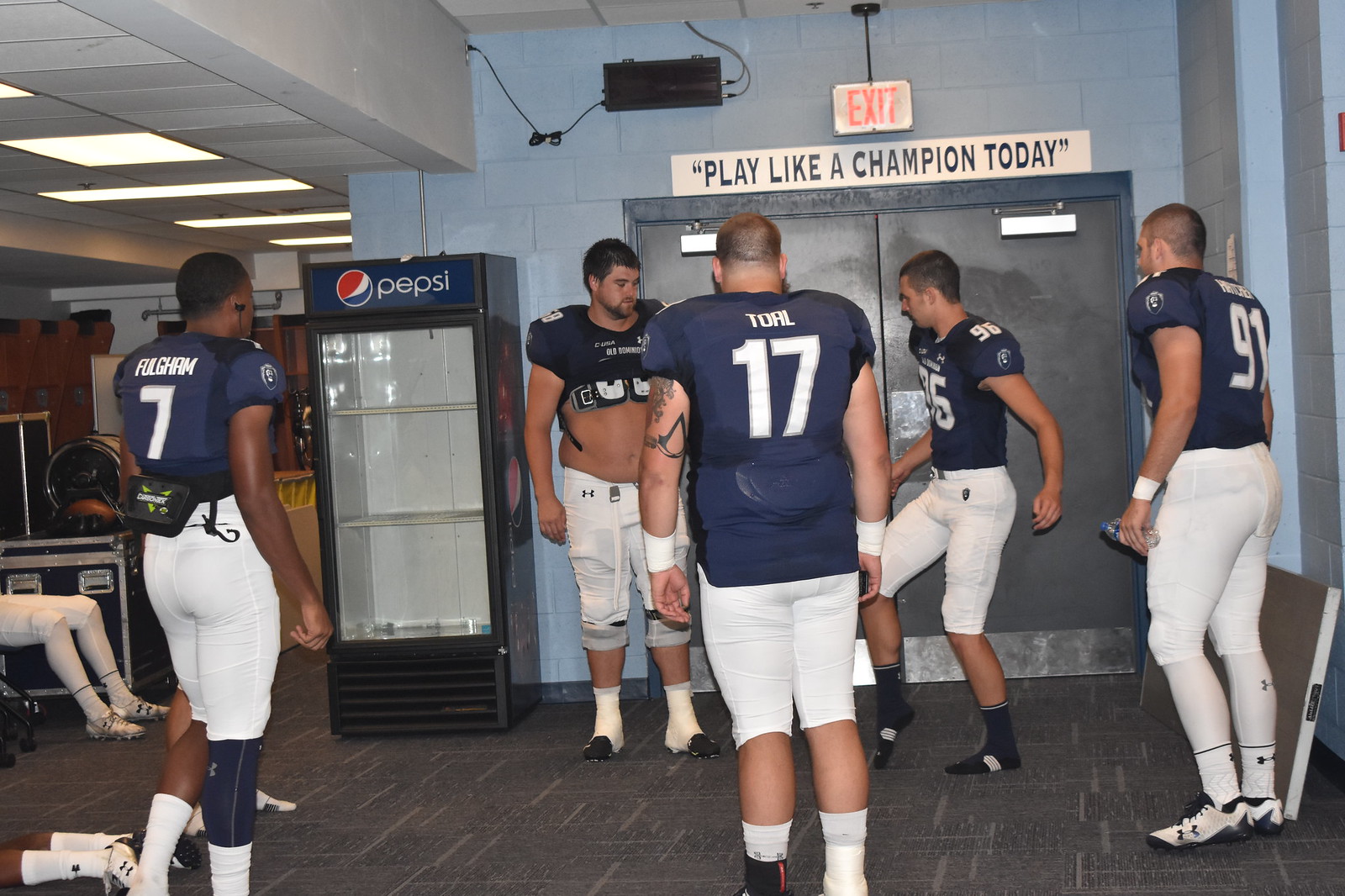This image captures five football players in a locker room, dressed in dark blue shirts and white shorts. Some players have white leggings on, while others are bare-legged. One player has his shirt pulled up above his chest. The players appear to be engaging in a hacky sack game, with one man poised to kick and another watching his foot. The diverse group comprises four Caucasian men and one African-American man. The players stand on a gray carpeted floor, surrounded by features such as a couple of double doors behind them, above which a white banner reads "Play Like A Champion Today" in black letters. Additionally, the room has recessed fluorescent lighting on the top left and a Pepsi vending machine. In the periphery, you can see parts of other individuals; someone’s legs are visible, seated on the left, and another player's feet sticking out as they lie on their stomach.